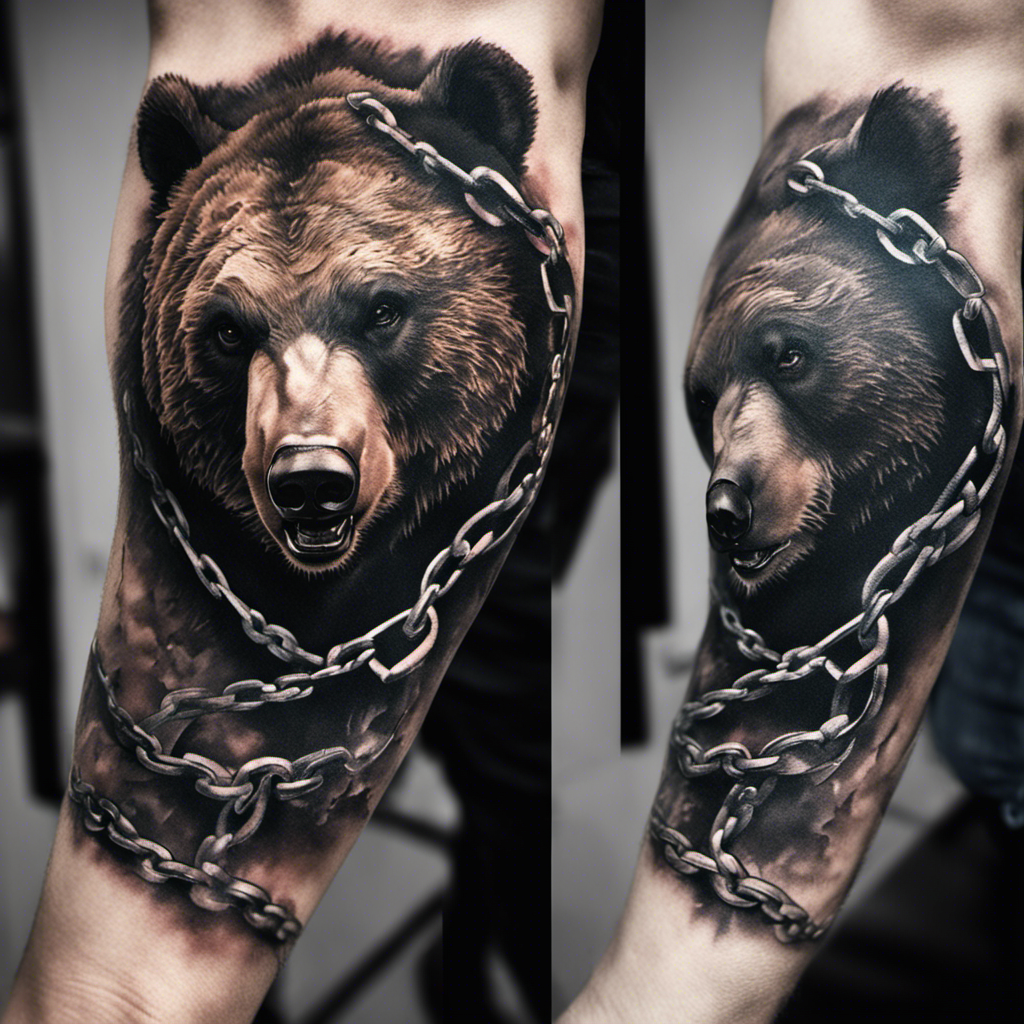This image features side-by-side photos of a detailed tattoo on a person's limb, potentially an arm or a leg. The tattoo showcases a realistic depiction of a grizzly bear, with the bear facing forward in one view and to the left in another. The bear's coat is dark brown with lighter inner parts, and it has a prominent black nose. A steel chain wraps around the bear's neck, looping around the chest and extending down the limb. The background of the image is gray with black shadows, emphasizing the intricate design and shading of the tattoo.